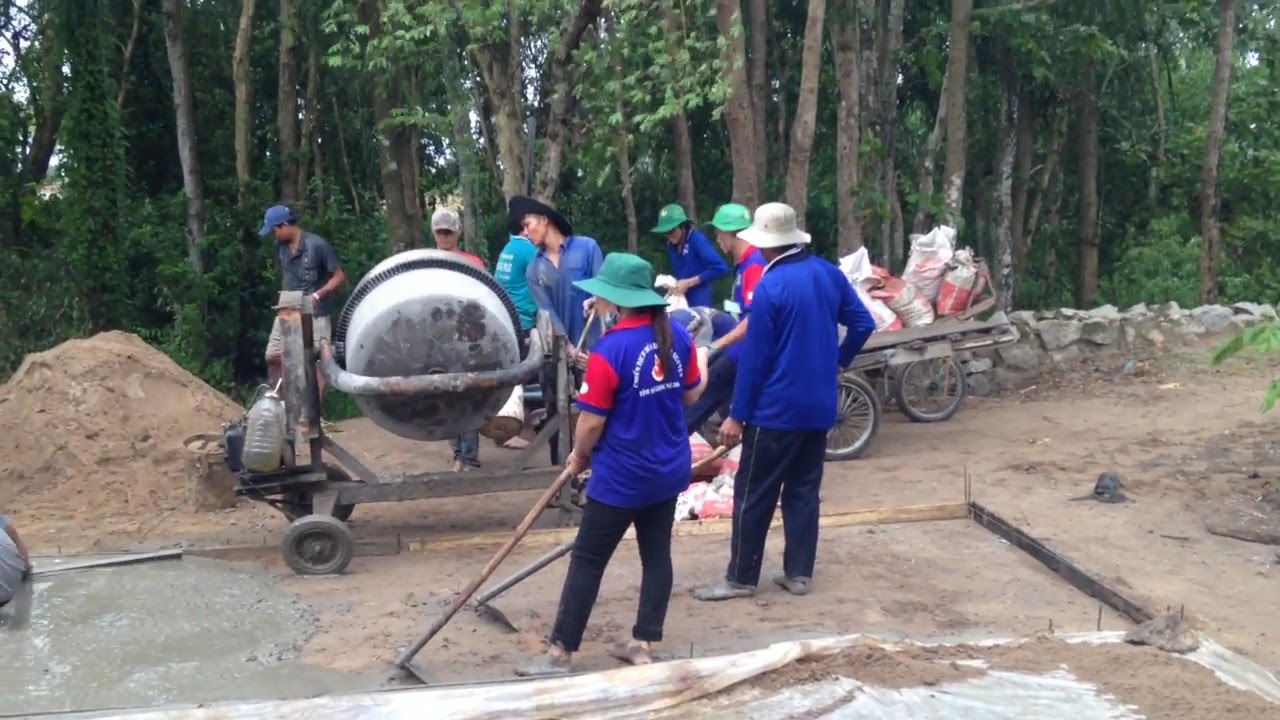This image captures a bustling group of approximately eight adults engaged in a construction project amidst a verdant background of medium to thin tree trunks and dense foliage, with hints of sky peeking through. The majority of the individuals are wearing bucket hats—predominantly green, with one white and one black—while a man on the left sports a blue baseball cap. It's a diverse scene with some participants clad in blue and red clothing, possibly indicating a volunteer effort, as they appear focused on laying the foundation for a new structure.

A woman and a man, both in blue pants and the woman in a blue shirt accented with red and white lettering, are seen in front, barefoot and working diligently to spread fresh cement with scrapers and a hose. The boxed area under construction is partly filled with concrete, delineated by wooden boards. Around them, there's an array of tools and equipment: a large cement mixer with a white drum on the left side, a pile of dirt, and a wagon loaded with bags likely containing cement, positioned towards the right.

The scene is lively, with some participants mixing concrete in the background, evidenced by the scattered bags of cement and a large mixing container. Their feet are caked in mud and concrete, emphasizing their hands-on engagement in this laborious task. The entire tableau is set against a backdrop of lush trees, adding a natural touch to the industrious atmosphere.